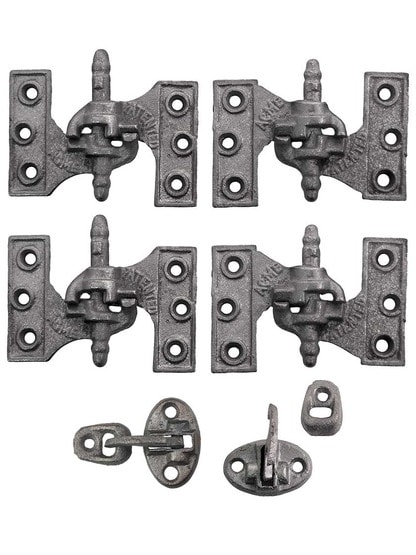The image features a collection of dark gray, metallic fasteners and hinges against a white background, likely die-cast metal. At the top are four identical door hinges with a rectangular form and three rivet or screw holes on each side for fastening, arranged in two pairs. These hinges have a central curved area where a single pole locks the two parts together. The word "Acme" appears overlaid on these hinges. Below these, there are three individual locking latches, distinct from each other. These latches are simpler in design, characterized by oval shapes and a latch mechanism that hooks into an opposing piece. The objects are likely door-related hardware, carefully positioned for the photo, which appears to be taken from above.